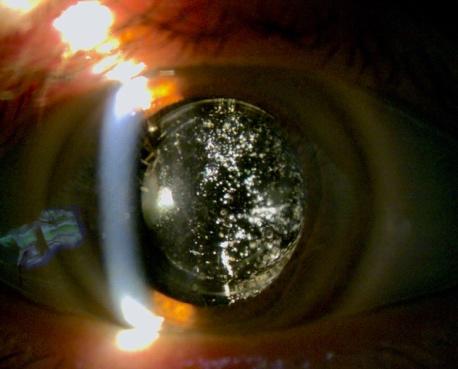The image appears to depict a close-up, artistic representation of an eye. The central focus is the dark, glassy iris that is almost black, interspersed with numerous tiny reflective white specks, resembling a piece of glass. Surrounding the iris are the whites of the eye, which have a yellowish tinge, and the eyelids that curve around the top and bottom, accompanied by distinctly pink eyelashes. To the left of the iris, there's a cloudy white line intersected by a bright light, possibly indicating a disease or a laser scanning the eye. The backdrop of the image is dark chocolate brown on the right, transitioning into a fiery red hue on the left, where a blue, candle-like object emits light in various directions, adding to the dramatic contrast and vivid color scheme of the painting. There's a blurred signage at the bottom, reinforcing the notion that this is an artistic piece rather than a straightforward photograph. The overall composition is intricate and evocative, blending detailed realism with abstract elements.